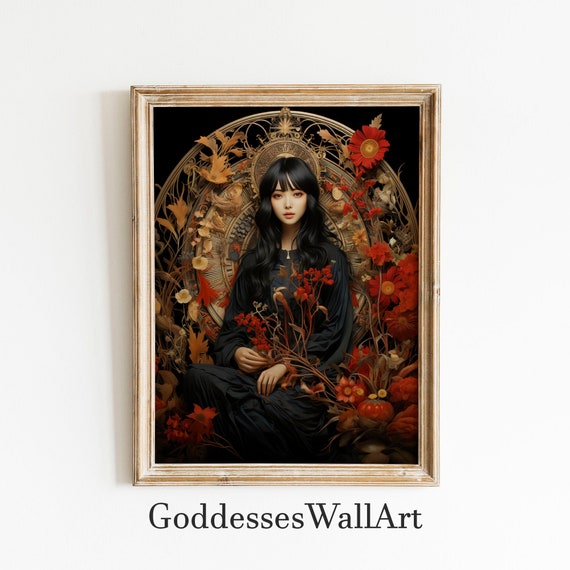Here is a cleaned-up and detailed caption for the image described:

---

This exquisite art piece, titled "Goddesses Wall Art," is displayed in a light brown wooden frame that has a textured, inward-tapered design. Set against a pristine white wall, the artwork features an Asian woman with dark hair and very light porcelain skin at its center, exuding an air of serenity and grace. The woman, elegantly dressed in dark clothing, is adorned with a necklace and is portrayed in a squatting pose, resting on her knees. Surrounding her are lush red roses that spill over into her lap, creating a vivid contrast against her attire and complexion. The backdrop is a gilded, circular design intricately embellished with gold filigree, which enhances the ornate nature of the piece. Additional red flowers, each with vibrant orange and yellow centers, accentuate the artwork's rich color palette. The background remains dark, further highlighting the striking elements of the composition.